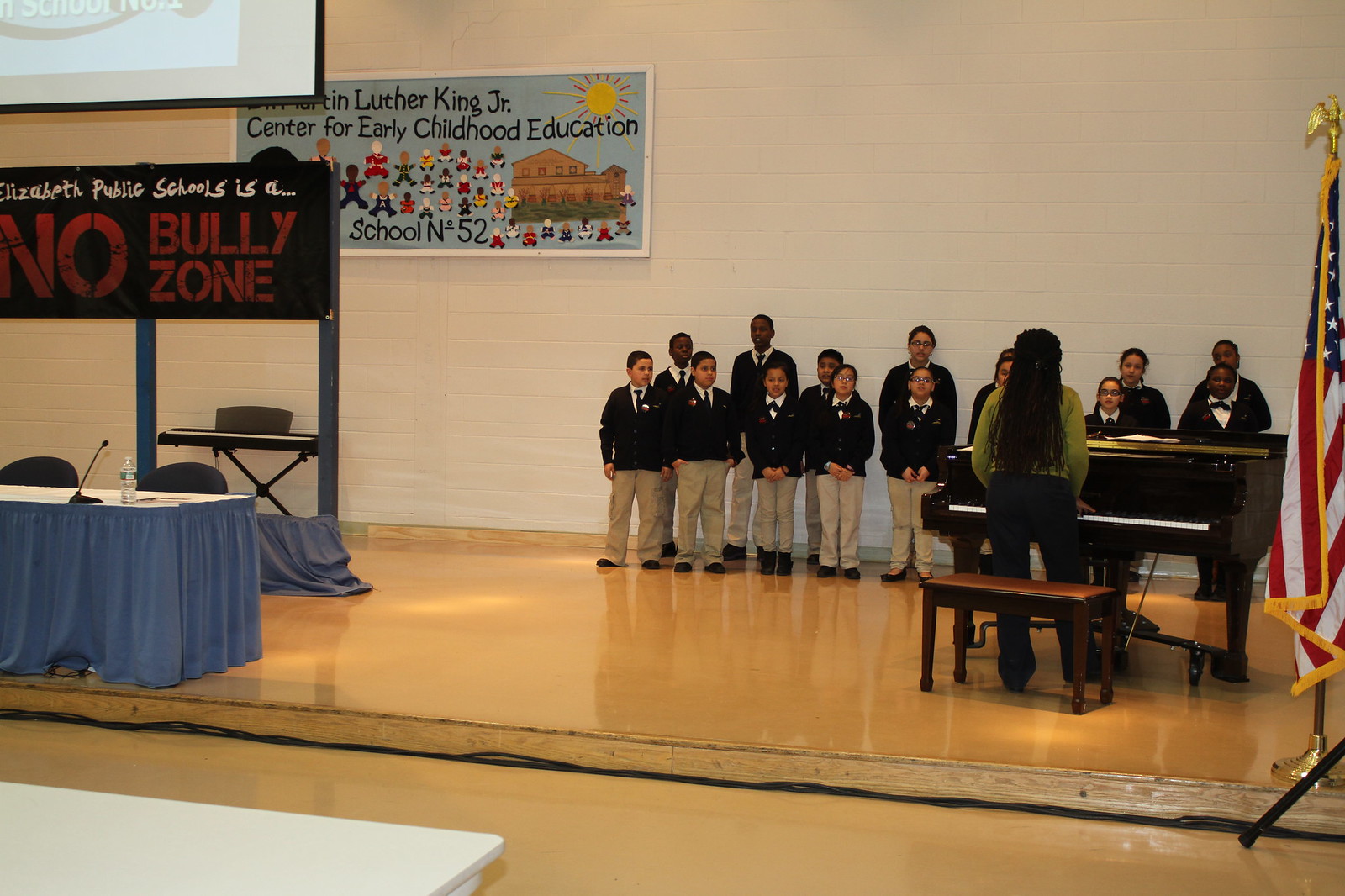The image captures a group of young children in school uniforms—comprising dark cardigans, white collared shirts, dark ties, and khaki pants—lined up in two rows. They appear to be part of a choir, standing on what seems to be the floor of a gymnasium or a stage setting, flanked by a white wall. To their side, a woman with long dark hair, wearing a green sweater, stands and plays a grand black piano placed in front of a brown bench, with the children facing her, likely singing. Behind the children, various elements are visible, including a cream-colored brick wall adorned with a poster featuring colorful cartoon images of children and a banner that reads "Luther King Jr. Center for Early Child Education." Additionally, signage includes "Elizabeth Public Schools is a no bully zone" and "school number 52." An American flag on a flagpole is partially visible on the right side, and an overhead projector casting an image is discernible in the background. A table with a blue skirt, a water bottle, and a microphone is positioned on the left.